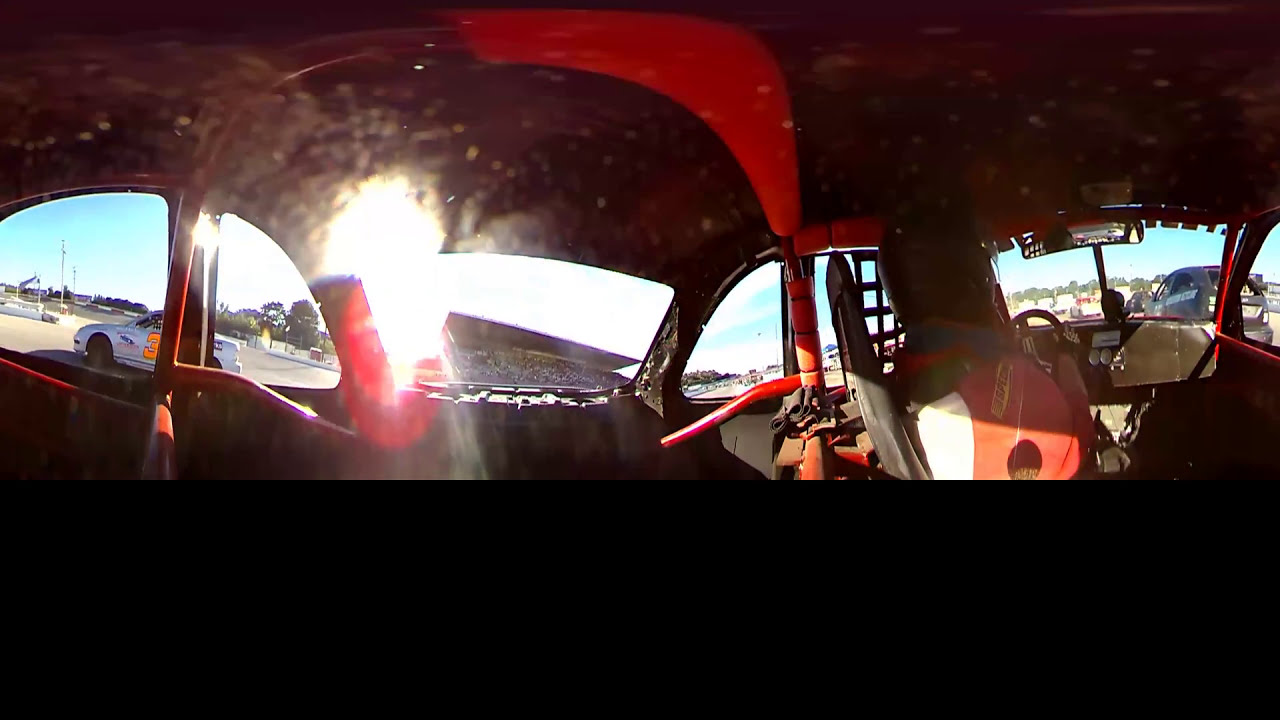This photograph captures the interior of an amateur race car taken from a backseat perspective, showcasing a panoramic view that includes both the driver and the surrounding environment. The driver, clad in a red racing jacket and black helmet, is seated in a thin black racing seat, securely strapped with black seat belts. He grips a black racing wheel and sits before a large, rectangular rear-view mirror. The interior of the car features a noticeable roll cage with orange padding and webbing, indicative of safety measures typical for racing vehicles.

Outside the car, under a sunny, bright blue sky, a variety of other vehicles can be seen on what appears to be a long and spacious racetrack. To the driver's right, a black van is visible, while on his left, a prominent white race car sports a bright neon orange number three. Surrounding the track, a grandstand filled with spectators adds to the vibrant atmosphere. Despite the dynamic setting, the image appears somewhat distorted, likely due to the 360-degree panoramic capture, offering a comprehensive view that includes the rear and side windows of the vehicle. This broad perspective also affords a glimpse of the sky and other elements outside, enhancing the detailed depiction of this racing moment.